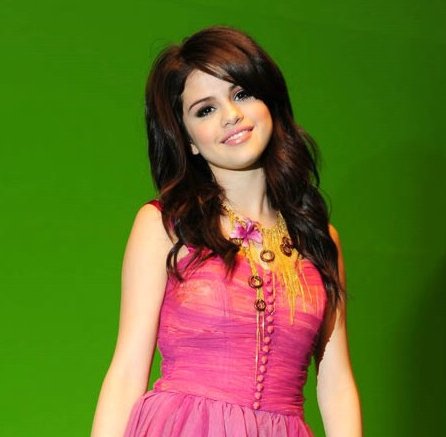This is a detailed portrait of Selena Gomez standing in front of a green background. She is wearing a vibrant pink, form-fitting dress with a pleated, textured skirt and numerous pink buttons running down the bodice. The dress is sleeveless with straps on the shoulders and features a visually artistic top with a draped effect at the bottom. Selena's long, thick, dark brown hair, slightly curly, cascades down past her shoulders to her chest. Around her neck is an ornate, yellow necklace adorned with rings, a pink flower, and yellow dangling strands, adding an extra touch of elegance. She stands slightly angled to the right, with her arms down by her sides, her head tilted to the left, and a warm, engaging smile on her face as she stares directly at the camera.